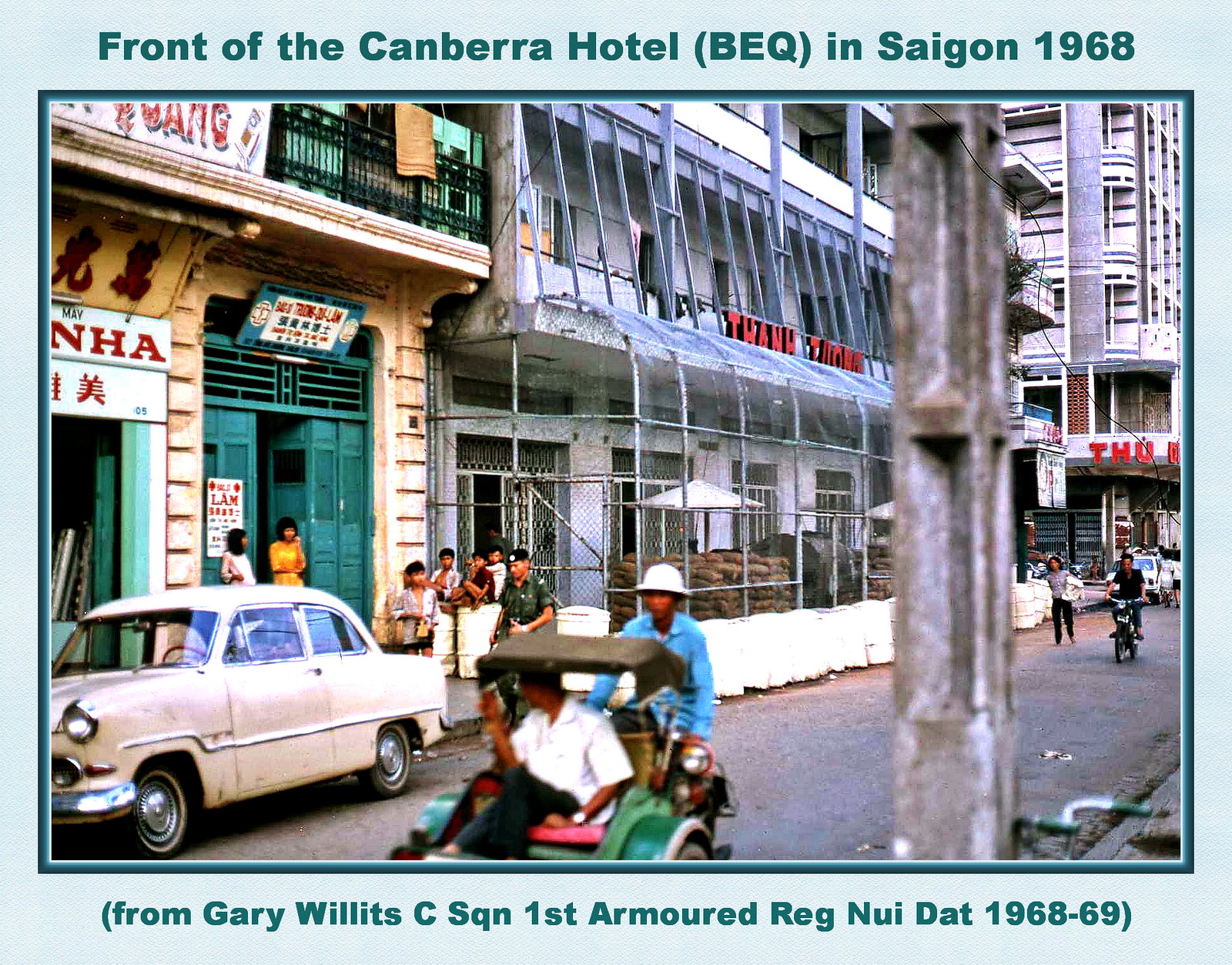This image is a detailed, photorealistic postcard depicting a bustling city street in Saigon, Vietnam, circa 1968. The street, which starts from the bottom left and leads to the right, features a variety of vehicles and pedestrians. In the foreground, a blurry rickshaw with a cloth roof is noticeable, along with some parked cars. On the sidewalk and further in the background, people are walking and riding bikes as motorcycles can be seen weaving through the street. The street is lined with a mixture of run-down and under-construction buildings. Notably, on the left side, there’s a white-bricked building with green windows and doors, while its neighboring building has a prominent red sign reading "Tan Tong" and is enclosed by a large fence. The buildings suggest a mix of commercial activities and possibly some military presence, as indicated by the sandbags and reinforced metal framework on one of the patios.

The image is framed within a light blue border, and at the top, dark green text reads "Front of the Canberra Hotel (BEQ) in Saigon 1968." At the bottom, similarly styled text states "From Gary Willett's C Squadron, 1st Armored Regiment, Nui Dat, 1968 to 69." This caption transforms the photograph into a historical memento, capturing a vivid snapshot of daily life during a turbulent period, likely intended for commemorative purposes.